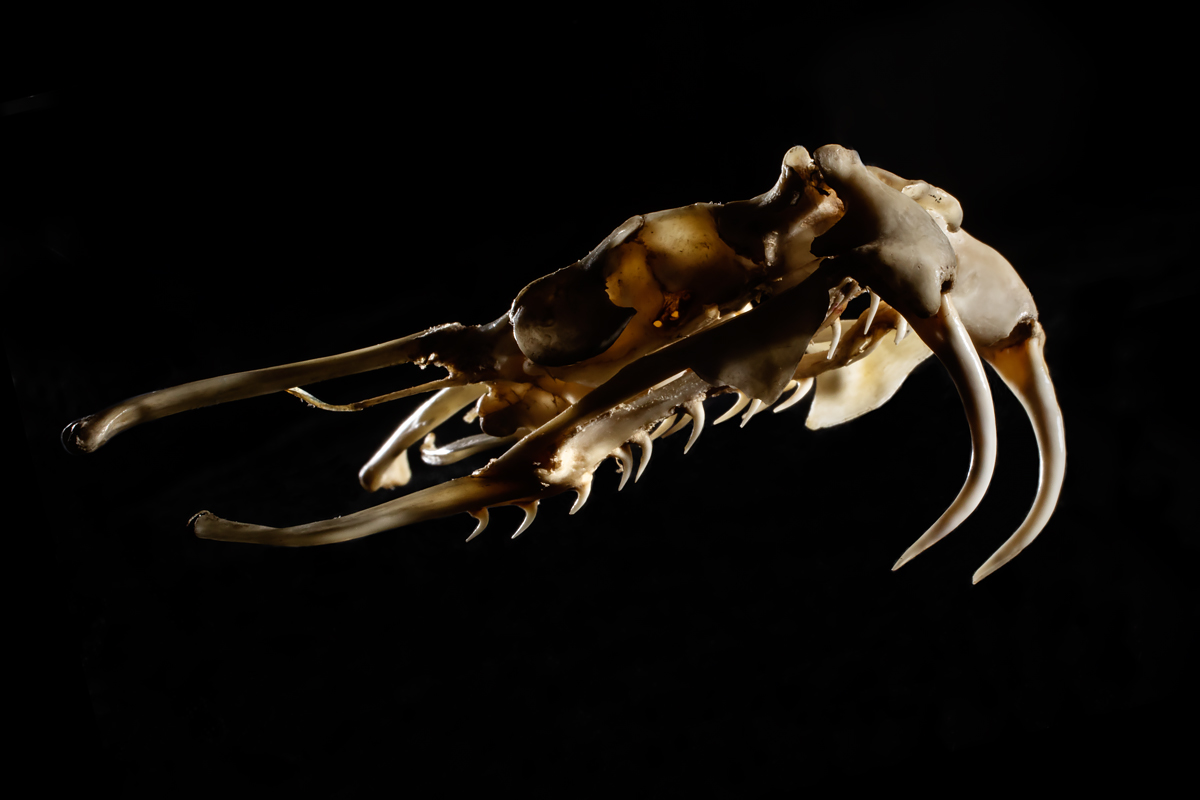The photograph features an off-white, possibly skeletal structure of indeterminate origins set against a solid black background. Dominating the center of the image, this ambiguous form resembles a skull but lacks clear identifying features such as eye or nostril sockets. The structure is equipped with two prominent prong-like projections extending from the front, and another pair arched downwards from the rear, curving to the left. There are additional thin, leg-like appendages protruding, marked by greenish-orangey tones and darker patches, suggesting they might be legs or part of the skeletal framework. Notably, the front displays fang-like elements and rows of what appear to be curved teeth, adding to its cryptic nature. The exact identity remains elusive, provoking curiosity as to whether this is the skull of an unfamiliar animal or simply another section of bone, possibly even an exoskeleton of an insect or a crab-like creature.